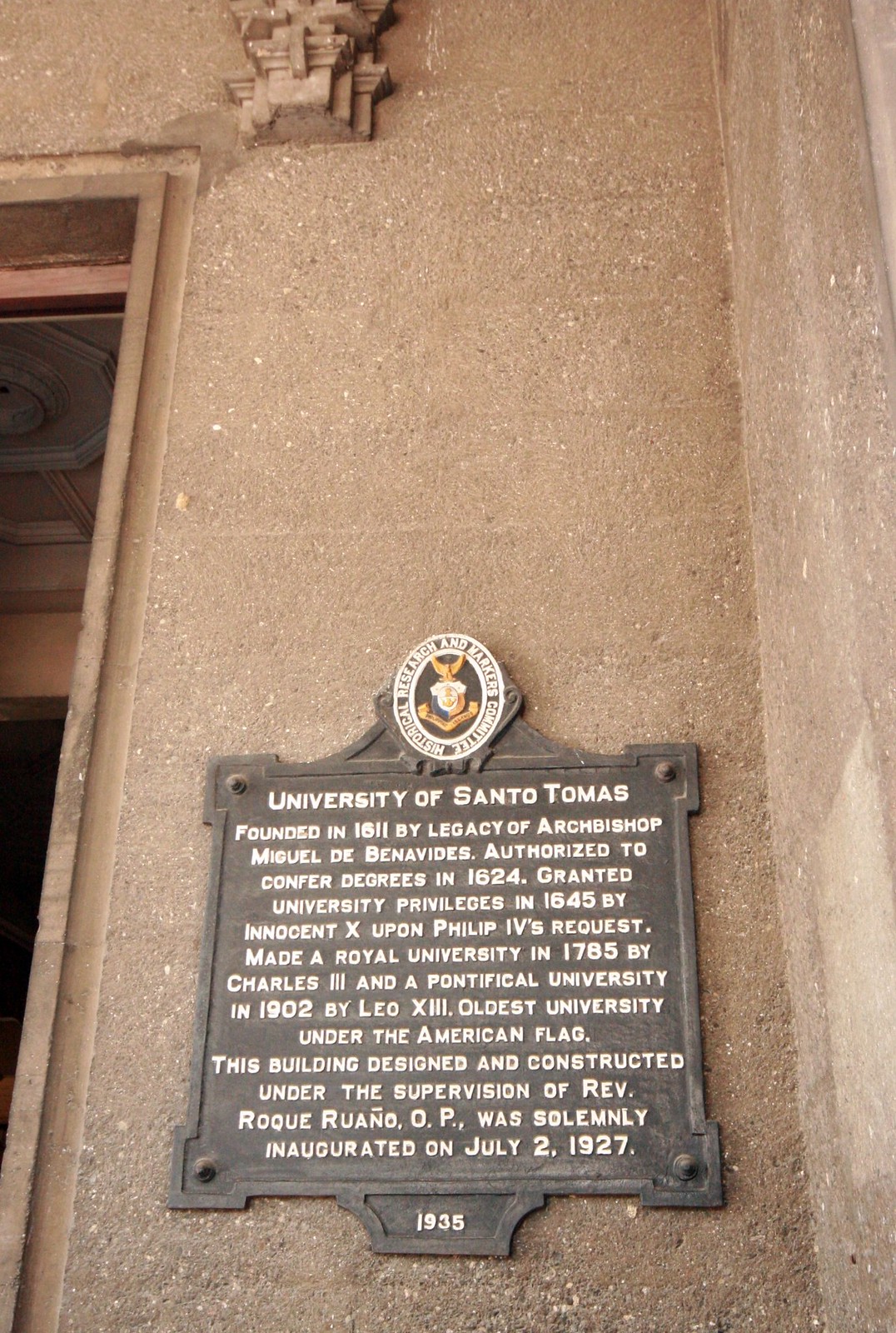This image showcases a metal plaque, possibly iron or brass, mounted on a concrete wall of a very old building. The plaque has a black background with white text and features an emblem at the top, surrounded by the words "Historical Research and Markers Committee." The emblem includes a coat of arms with a bird atop it. The detailed inscription on the plaque reads:

"University of Santo Tomas, founded in 1611 by the legacy of Archbishop Miguel de Benavides, authorized to confer degrees in 1624, granted university privileges in 1645 by Innocent X upon Philip IV's request. It was made a Royal University in 1785 by Charles III and a Pontifical University in 1902 by Leo XIII, making it the oldest university under the American flag. This building was designed and constructed under the supervision of Reverend Roque Roanio, OP, and was solemnly inaugurated on July 2, 1927. This plaque is dated 1935."